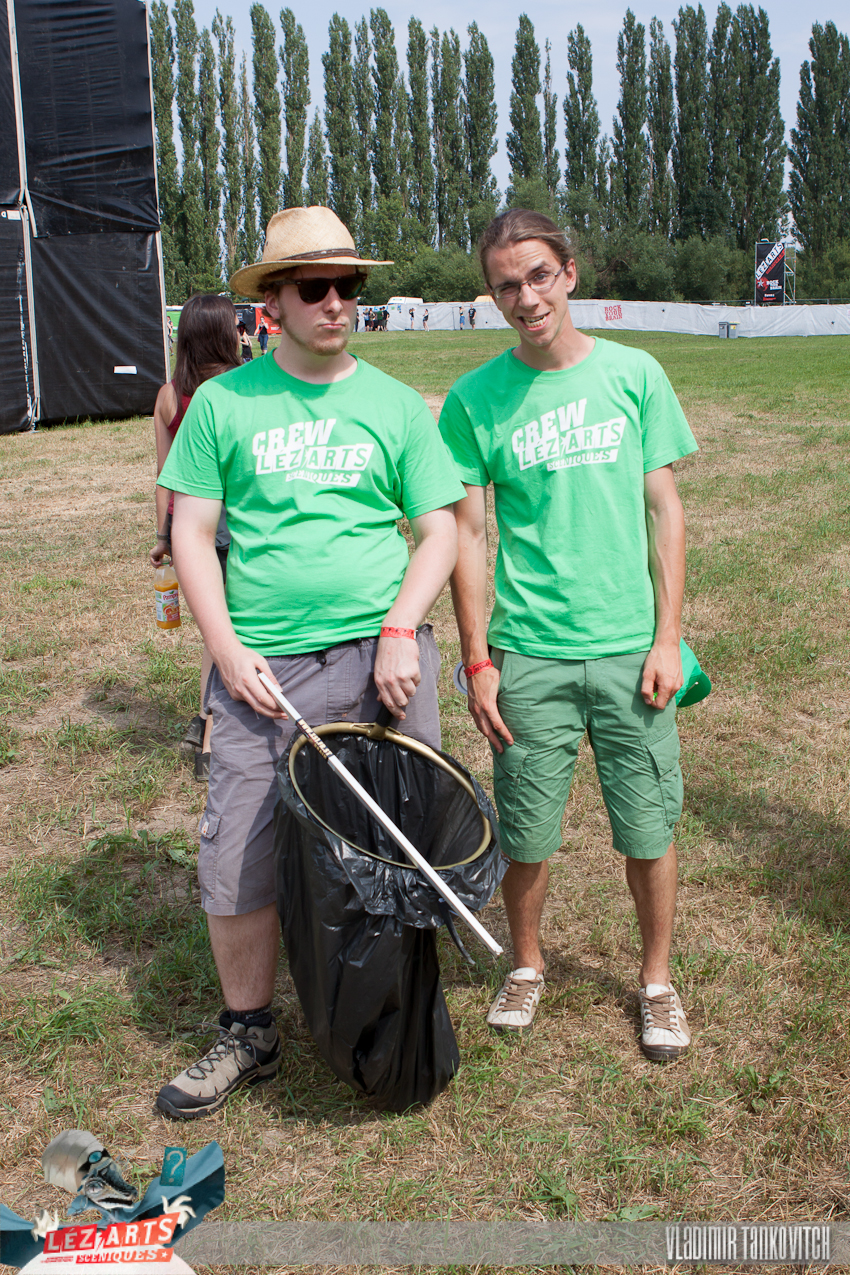In this outdoor photo, two men stand on a field of predominantly brown, drought-affected grass with some patches of green. Both wear green shirts emblazoned with white letters reading "Crew Lazarts". The man on the left, who sports sunglasses and a tan brimmed hat, is holding a trash bag with a circular rim in one hand and a litter pickup stick in the other. He also wears gray cargo shorts and a red wristband. The man on the right, with his hair tied back and wearing regular glasses, is clad in darker green cargo shorts, also paired with a red wristband. Behind the man on the left, a woman with dark hair holds what appears to be a juice bottle. The background reveals a large structure covered in black tarps, tall trees, and a white-bordered fence with advertising. In the lower left, there's an indistinct green object on the ground and a red logo with white letters spelling "Les Arts." The photographer's name is faintly visible in white in the lower right.